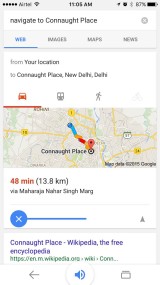This image is a screenshot captured on a cell phone with a light gray background. At the top of the screen, there are five black-filled dots indicating signal strength, and next to them, the blurry text appears to say "Airtel." This is accompanied by a Wi-Fi signal icon, and the time is displayed as 10:00 AM. To the left, there are small icons for Bluetooth, an alarm, and a battery indicator showing 87% with a battery icon.

Beneath this, there is a search bar displaying the text "Navigate to Connaught Place," with a round gray circle containing an 'X' on its right side. Following the search bar, there is a navigation menu with options reading "Web," "Images," "Maps," and "News," these are highlighted in blue and underlined.

A white banner below the menu reads, "From your location to Connaught Place, New Delhi, Delhi," showing transportation options with a red car icon that is underlined, along with bus and walking icons. Below this, a map is visible highlighting Connaught Place with a location tag.

Under the map, a white banner states it will take "48 minutes" in red text, followed by the distance in parentheses as "13.8 KM." Toward the bottom of the screen, there is a line featuring a blue circle with an 'X,' continuing to "Connaught Place, Wikipedia, the free encyclopedia," along with its website link.